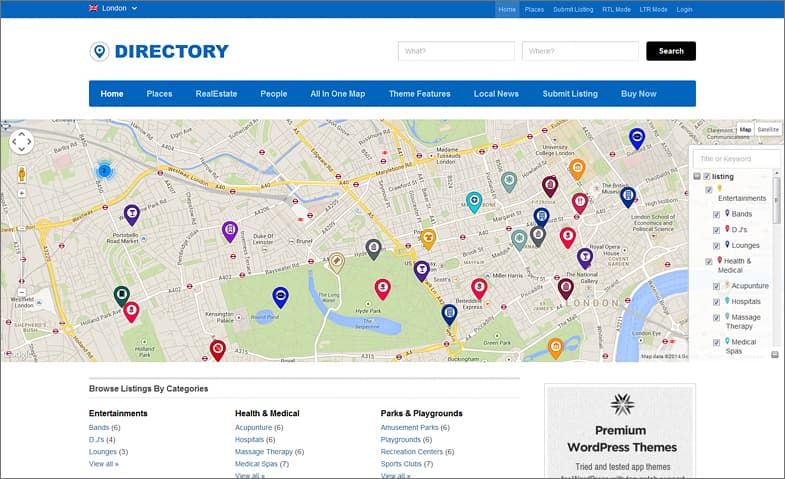This is a detailed caption for the image described:

---

The screenshot depicts a comprehensive online directory for London, prominently featuring a navigation header at the top. The header contains the word "London" alongside a red, boxy graphic with illegible text. On the right, "Directory" is displayed in bold blue letters accompanied by a blue pin icon. The interface includes two search bars labeled "What" and "Where" with a black "Search" button. Beneath this are various navigation options highlighted within a blue border: "Home," "Places," "Real Estate," "People," "All in One Map," "Theme Features," "Local News," "Submit Listing," and "Buy Now."

Central to the image is a large, detailed map with multicolored pins (including purple, red, blue, yellow, and peach) indicating various locations. To the right of the map, the word "Listing" is displayed, followed by a key, another search bar, and categorized listings such as "Entertainment," "Health and Medical," and "Massage Therapy." Moreover, several services are noted, with their respective pins visible on the map.

Further below, under the "Browse Listings by Categories" section, categories including "Entertainment," "Health and Medical," and "Parks and Playgrounds" are listed. In the lower right-hand corner, a gray box advertises "Premium WordPress Themes."

---

This caption highlights the key elements and navigational features of the directory website, providing a clear understanding of its layout and functionality.